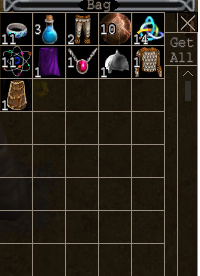The screenshot depicts a pixelated inventory screen from what appears to be a late 90s or early 2000s role-playing video game with a nostalgic feel reminiscent of titles like Dungeon Siege or Dungeons and Dragons. The background is a dark brown to black with a five-column by nine-row grid, though only the top three rows contain items. The top border features a gray bar labeled "BAG" in white letters, and the right border includes an "X" for closing the inventory and a "GET ALL" button beneath an upward-pointing arrow, indicating items available for collection.

In the grid, various items are displayed along with their quantities: 
- The first square on the top row contains 11 rings.
- The second square holds 3 potions.
- The third square features 2 pairs of pants.
- The fourth square shows 10 shields.
- The fifth square contains 14 triskelion symbols in blue and yellow.

On the second row:
- The far-left square displays 11 atom symbols.
- The second square has a single purple cape.
- The third contains a red and silver necklace.
- The fourth shows a silver helmet.
- The fifth square holds a silver chest piece.

The third row:
- The first square on the left contains 1 brown cloak.
- The remaining squares are empty.

This is a detailed inventory view displaying the diverse items a player has collected in the game, such as wearable equipment, symbols, and consumable potions.